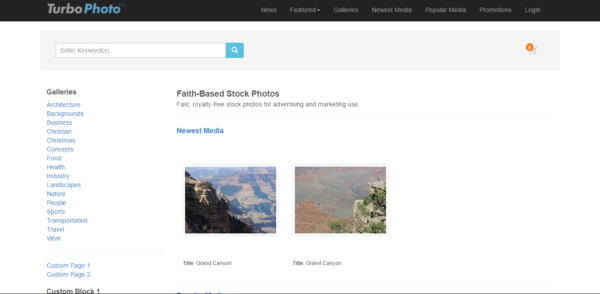This is a detailed description of an image showing a screenshot of a website that is wider than it is tall. The screenshot captures only the webpage content, excluding any browser window or borders. 

At the top of the page, there's a black banner stretching horizontally. On the left side of this banner, the website's logo reads "Turbo Photo" with "Turbo" in gray and "Photo" in blue, slightly indented to the left. Beneath this banner, there is a gray box. On the left side of this gray box, there is a white search bar with a blue search button featuring a magnifying glass icon on its right side. 

Toward the far right of the gray box, there's a shopping cart icon with a small orange circle, though the contents of the cart are not discernible. Below the gray box, the page has a solid white background.

On the far left side of this white section, there's a column labeled "Galleries." Under this label, multiple blue text links are listed line by line in a small font, including categories like "Architecture," "Background," and "Business." Each piece of text is presumably clickable, although the small size makes them difficult to read clearly.

To the right of the "Galleries" column, there appears to be a section potentially related to faith-based stock photos, indicated by a small font description and a brief script below an image or title. 

Further down, an area titled "Newest Media" in a combination of white and blue fonts showcases two side-by-side outdoor photographs, reminiscent of landscapes such as the Grand Canyon.